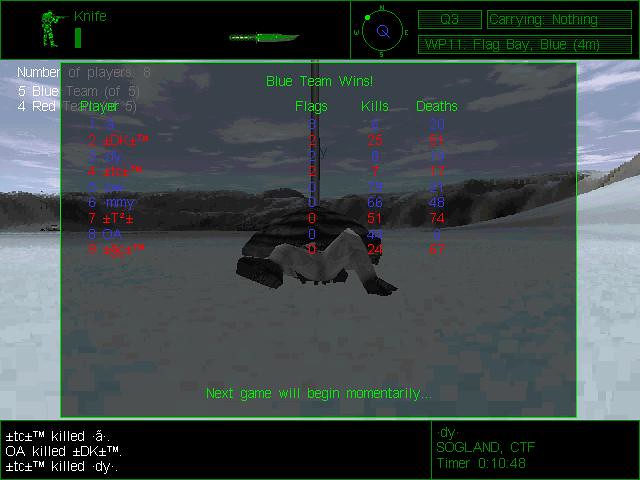This image is a screenshot from a video game. At the top, a black banner features green text and details. On the left-hand side, a character dressed in camouflage holds a gun. Next to the character, the word "Knife" appears with a corresponding knife icon to its right. The screen is divided, showing a compass in the middle. Below the compass, there are three green boxes containing information: "Q3," "Carrying Nothing," and "WP11 - Flag Bay Blue, 4 mm."

The background is gray, and centrally positioned is a score box indicating that the next game will begin shortly. It displays "Blue Team Wins" along with statistics such as scores, flags, kills, and deaths. At the bottom of the screen, another black banner displays a timer.